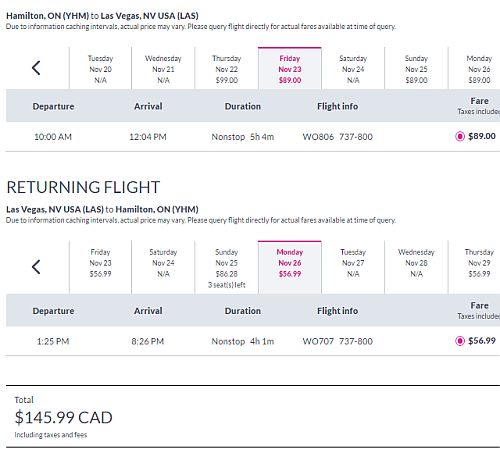This image displays flight information for a trip from Hamilton, Ontario (YHM) to Las Vegas, Nevada, USA. The image notes that due to information caching intervals, the actual prices may vary, and it advises querying flights directly for the most accurate fares at the time of booking. The flight availability and prices for specific dates are as follows:

- Tuesday, November 20th: Not available
- Wednesday, November 21st: Not available
- Thursday, November 22nd: $99
- Friday, November 23rd: $89 (selected day)
- Saturday, November 24th: Not available
- Sunday, November 25th: $9
- Monday, November 26th: $9

For the selected flight on Friday, November 23rd:
- Departure time: 10:00 AM
- Arrival time: 12:04 PM
- Flight duration: Non-stop, 5 hours and 4 minutes
- Flight number: W0707
- Aircraft type: W737-800-FE
- Base fare: $56.99